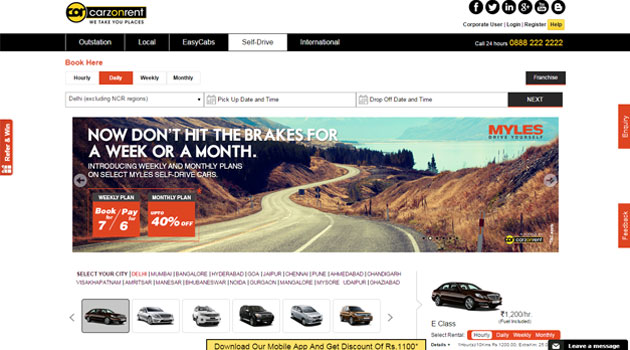This image depicts a car rental website interface, prominently featuring a sleek logo - a yellow circle with a black border containing the word "Car" in bold, black letters. A navigation bar at the top lists various options such as Customization, Local Rent, Easy Cabs, Self Drive, and International Services, though these labels are diminutive and challenging to read. The website proudly advertises 24-hour service with a contact number for around-the-clock assistance.

A call-to-action invites users to book online with flexible rental periods categorized into hourly, daily, weekly, and monthly rates, with the daily rate section highlighted in red for emphasis. The website displays a scenic image of a winding road flanked by rocky terrain, captioned with a motivational slogan: "Now don't hit the brakes for a week or a month. Introducing weekly and monthly plans on select Miles self-drive cars."

Two promotional offers are featured prominently: a 40% discount on monthly rentals and a "Book seven days, pay for six" weekly plan. The top-right corner of the site bears the brand name "Miles." Below the main image, users can browse images of available rental cars and are encouraged to download the mobile app for additional discounts.

An orange vertical line, with horizontal text alongside it, promotes a "Refer and Win" program, adding another layer of engagement for potential customers.